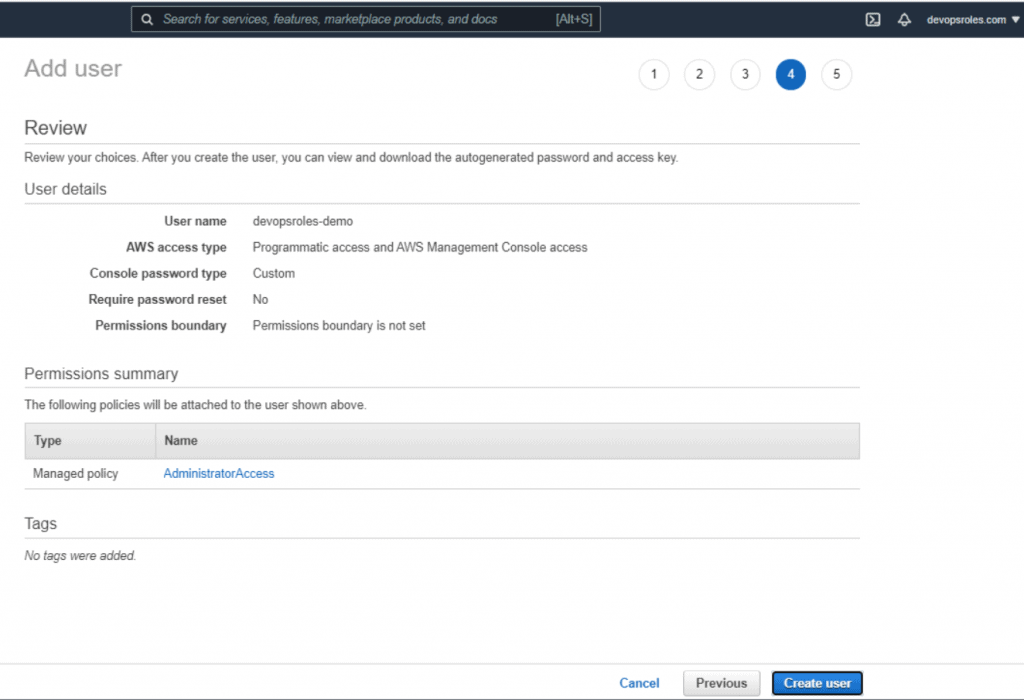In this image, we see a detailed user interface for a web service related to DevOps. 

- In the top right corner, the header displays the site name "DevoPSRoles.com" accompanied by a small white downward arrow.
- Adjacent to the site name, there is a bell icon and a square icon, likely representing notifications and settings, respectively. 
- Moving leftward, there is a search bar with placeholder text reading "search for services, features, marketplace products, and docs," and a shortcut hint (Alt + S) to the right.
- Below the header, in the top left, there's a light gray text that reads "Add User." Nearby, there are five numbered circles (1 through 5). The fourth circle stands out with its blue background and white number, indicating an active step in a multi-step process.
- On the far left, the text "Review" appears, signifying the current section of the process. Below this is a horizontal line followed by the phrase "Review your choices. After you create the user, you can view and download the auto-generated password and access key."
- The "User Details" section is located under another horizontal line and provides fields including "Username," "AWS access type," "Console password type," "Required password reset," and "Permissions boundary."
- At the bottom right, there are three buttons: "Create User," "Previous," and "Cancel," allowing users to finalize, revisit, or abort the process.

Overall, the image seems to capture a step in the user creation workflow within a DevOps platform, focusing specifically on reviewing and confirming user details before completion.